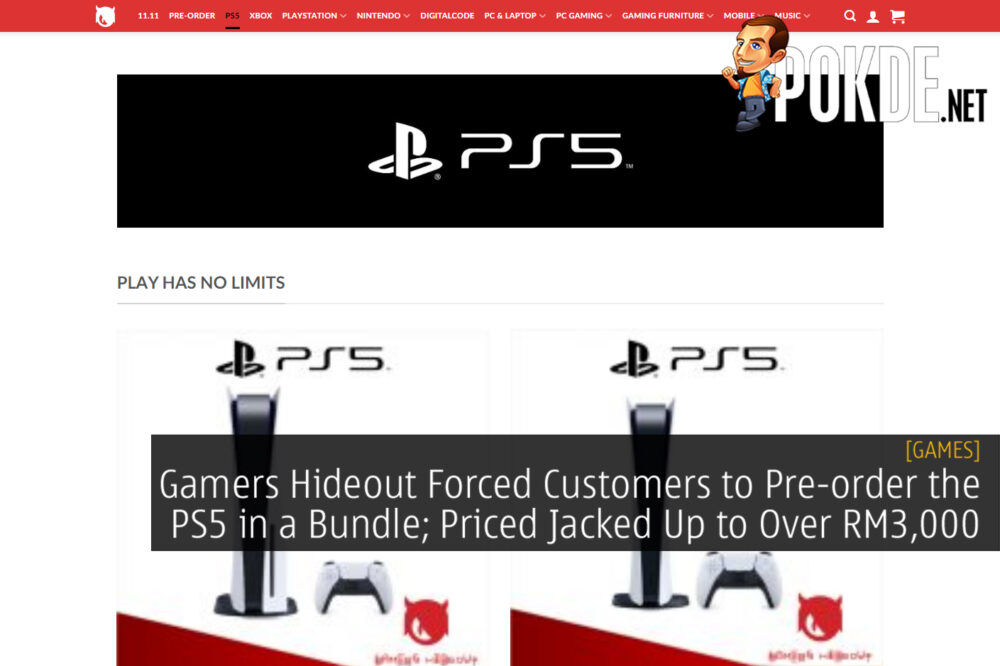The image showcases promotional content centered around gaming and electronics. At the top, a vibrant red bar highlights various categories including Xbox, PlayStation, Nintendo, digital codes, PC and laptop, PC gaming, gaming furniture, mobile, and music. Within this red banner is a white magnifying glass icon, a white user icon, and a white shopping cart icon.

Below this, the site name "Pokedepopd.net" is displayed with a small cartoon man leaning against the text, creating a playful visual element. Another prominent feature of the image is a black bar prominently stating "PS5," followed by the slogan "Play Has No Limits" and repeating "PS5" twice, emphasizing the product being advertised.

The lower section reveals a controversial note: "Gamers Hideout forced customers to pre-order the PS5 in a bundle, price jacked up to over RM3000," suggesting discontent over perceived unethical pricing practices. This image appears to be an advertisement with an underlying message pointing out questionable activities related to PS5 pre-orders.